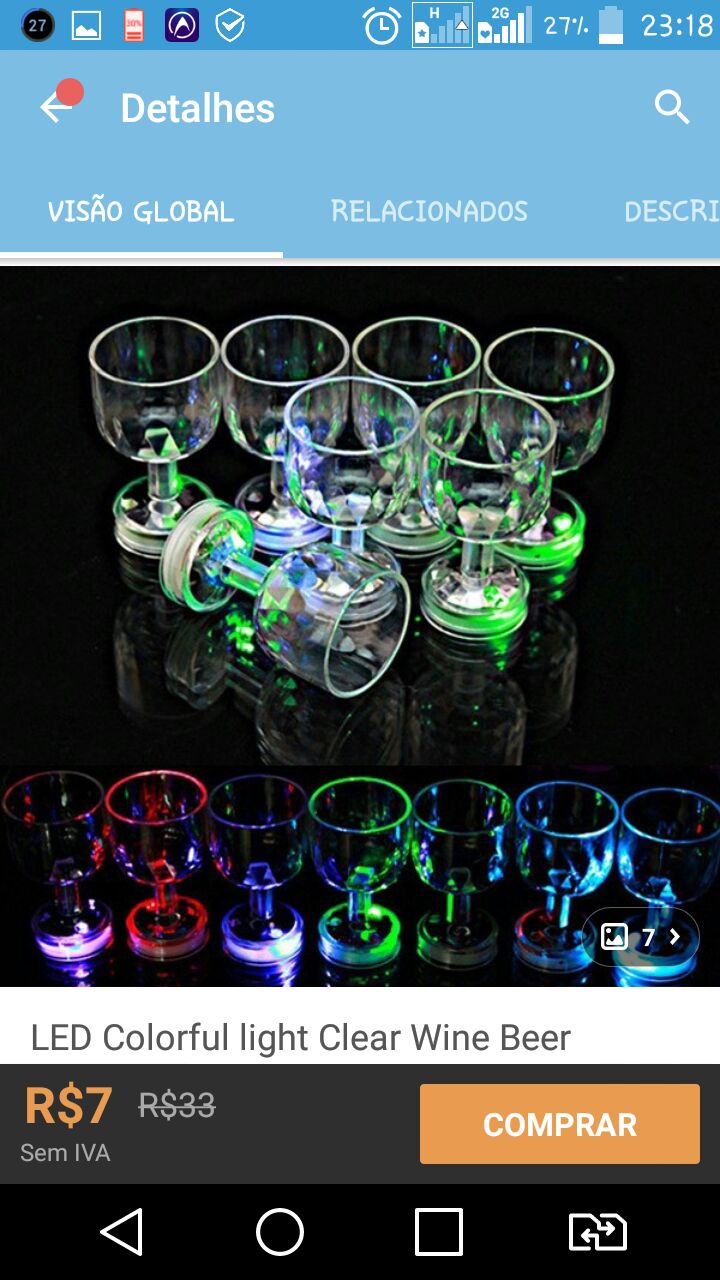This image depicts a screenshot taken from a smartphone, featuring an online listing of LED colorful light clear wine and beer glasses on a shopping website. The screenshot captures typical smartphone icons like battery life, time, cell signal, and wifi at the top right corner, indicating it was taken from a mobile device. The language on the phone appears to be Spanish or something similar, with symbols and text on a dark blue status bar at the top. Below, a lighter blue strip houses store-related information with a distinctive red dot on an arrow icon.

The main visual in the screenshot is an array of seven clear wine glasses, with the one on the bottom left positioned on its side. These glasses are illuminated by LED lights, causing them to shine in various colors such as red, blue, and green, producing an iridescent, neon effect against a black backdrop. At the bottom of the advertisement, the text “LED colorful light clear wine beer” is displayed in black. Additionally, there are four navigation icons at the very bottom, shaped like a triangle, a circle, a square, and an S-shape with arrows, which likely serve as directional buttons for the smartphone. The price is displayed in foreign currency, with an orange button labeled "Comprar," suggesting the shopping context.